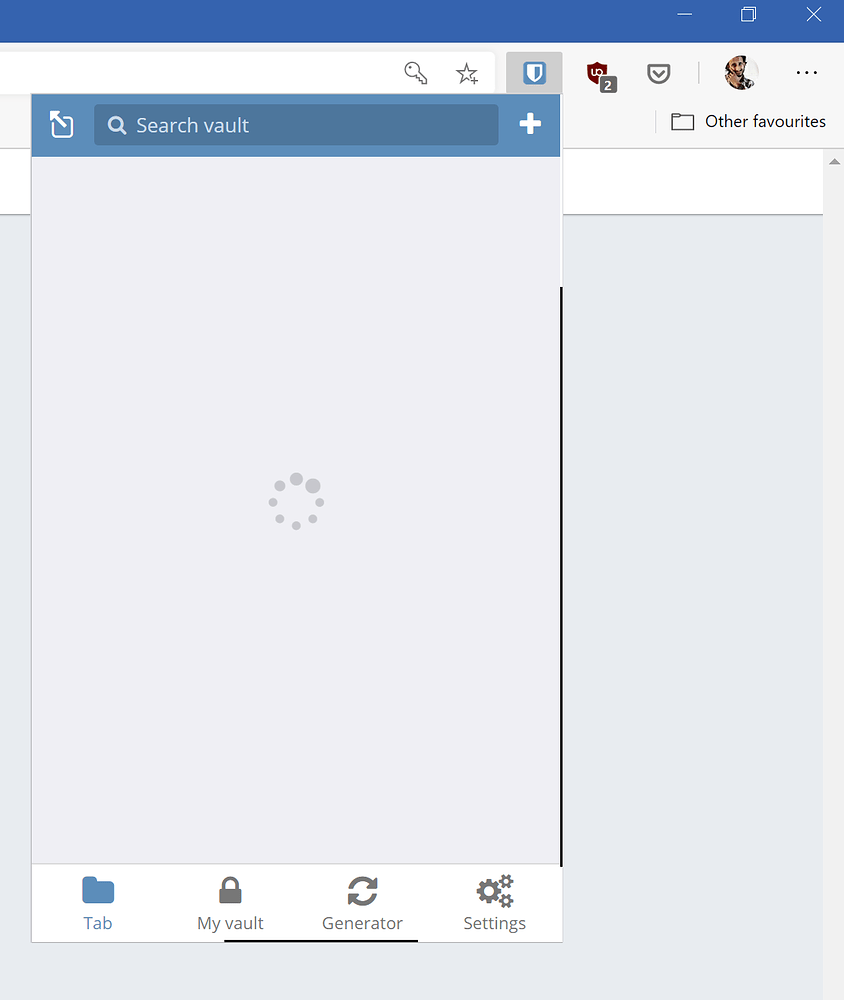This image showcases a computer screen displaying what appears to be a user interface, likely from a Windows-based application. The layout is divided into two primary sections: the top fifth of the screen features a white background, while the remainder is a very light gray. 

A blue title bar spans the top of the interface but contains no text. On the right side of this bar are the standard Windows controls: minimize, open a new tab, and close buttons. Below the title bar, a small pop-up window is visible. This pop-up contains a white rectangular area at the top housing several icons on the right: a key, a star with a plus sign, and a small, darker gray box with a blue shield icon, possibly indicating an ad blocker or security feature.

Directly below this white section is another blue bar. On the left side of this bar is an icon—a square with an arrow pointing up and to the left, likely representing a "send" or "share" function. Adjacent to this is a darker blue rectangle containing a magnifying glass icon and the text “search vault,” indicating a search function. Following this is a white plus sign.

The overall background of the main screen area is a very pale gray. At the bottom of the interface, the navigation options include tabs labeled "Tab," "My Vault," "Generator," and "Settings."